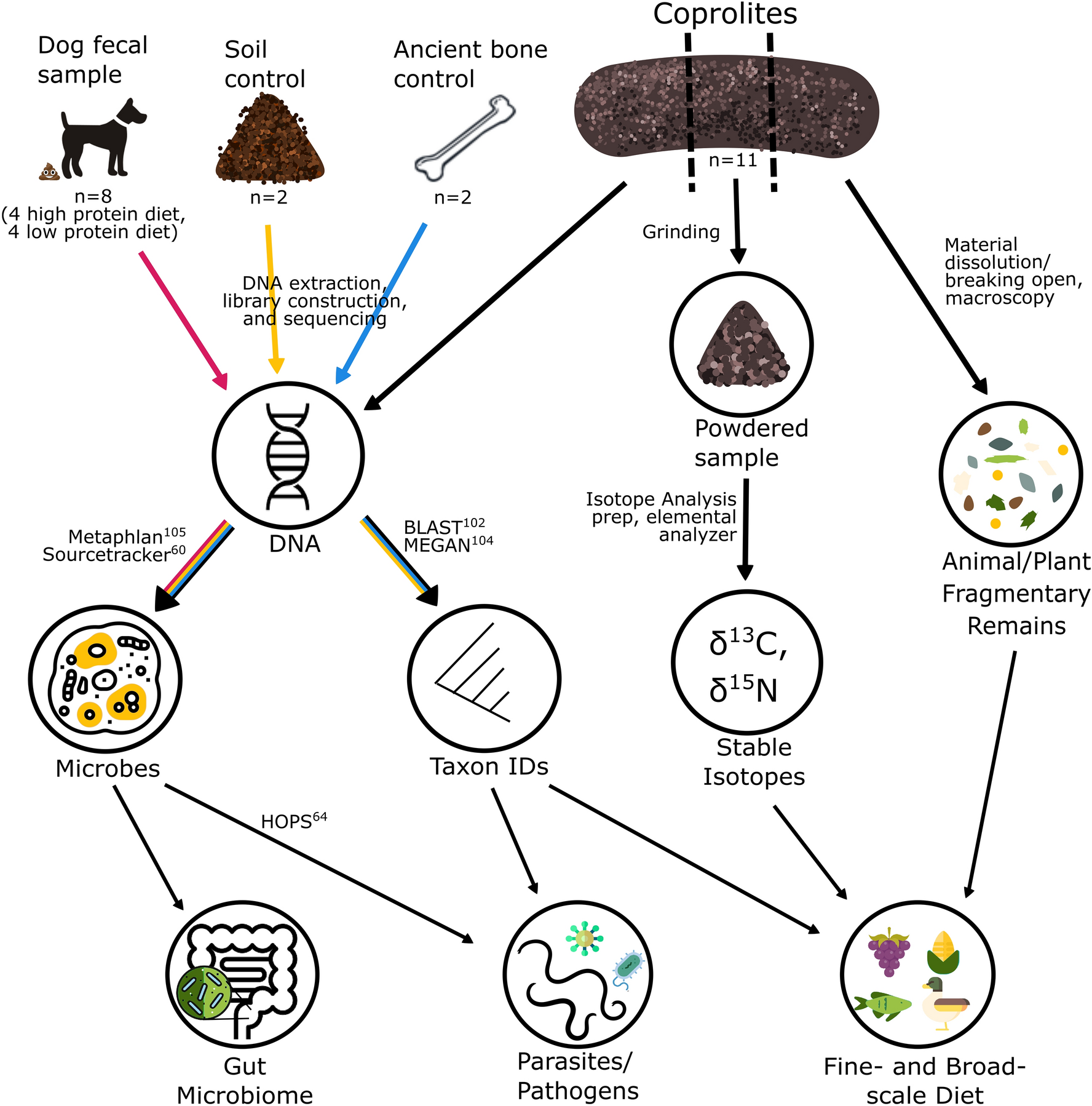The image is a detailed schematic diagram of a biological process involving dog fecal samples, comparing high-protein and low-protein diets across eight dogs. At the top, it labels three different control types: dog fecal sample, soil control, and ancient bone control, with icons depicting a dog (alongside a poop emoji) and other contextual elements. Arrows lead from each control to the stages of DNA extraction, library construction, and sequencing.

The diagram further illustrates the analytical process, with circles connected by arrows pointing to various components such as parasites, pathogens, the gut microbiome, and taxon IDs. It also includes references to both fine and broad-scale diet analysis, fragmentary animal and plant remains, stable isotopes, and powdered samples. Annotations mention the use of tools such as MetaPhlAn (Metagenomic Phylogenetic Analysis), SourceTracker, BLAST (Basic Local Alignment Search Tool), and MEGAN (MEtaGenome ANalyzer). The process highlights coprolites (fossilized dung), material dissolution, grinding, and macroscopy to denote the breakdown and examination of samples. Overall, the schematic provides an in-depth view of the microbial and dietary investigations conducted on the dog fecal samples.